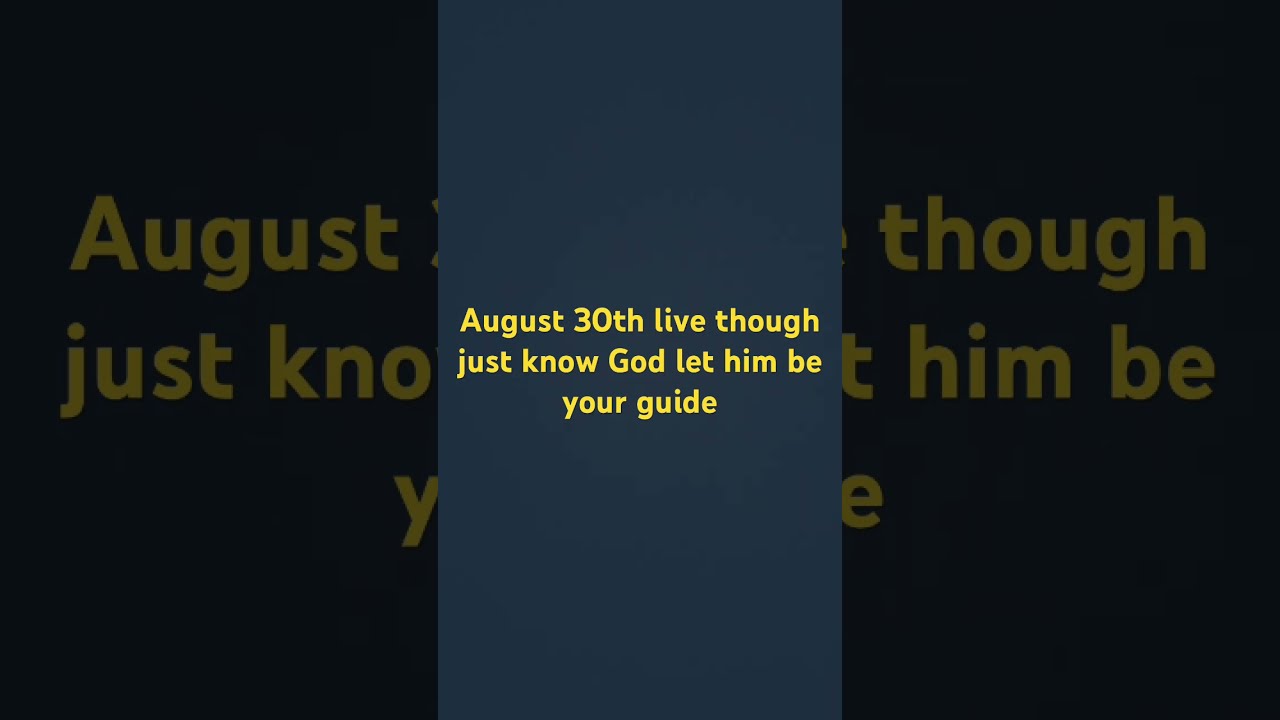The image is a vertically-oriented cell phone screenshot featuring a graphic with a dark, faded-gray background. Yellow text is centered from top to bottom within the image, and reads: "August 30th, live through, just know God, let him be your guide." The text appears three lines, layered one below the other and the screenshot is zoomed in, creating a blurred and darkened effect on both the left and right edges. Additionally, a dark blue vertical banner with the same yellow text partially overlays the center, repeating the message, "August 30th, live through, just know God, let him be your guide," but obscured by the zoom effect around the edges.